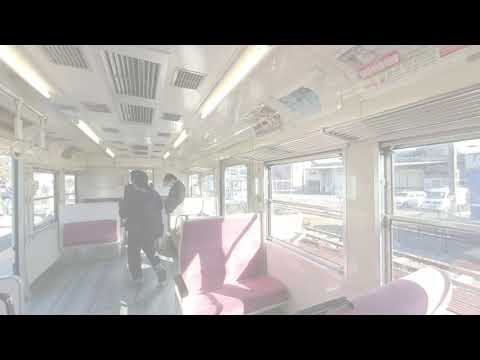The image is heavily overexposed, washing out most colors and making the overall scene appear overly bright. Occupying the center are two individuals standing inside what seems to be the interior of a train or subway car, indicated by the long, narrow structure with seats facing each other. The person in the middle partially obscures a passage to another car, while the other stands slightly to the right. The scene includes red-cushioned seats, although the exposure makes their true color hard to discern. The image has black borders at the top and bottom, and the setting seems to be a stopped train at a station during the day. Various colors such as black, white, grey, yellow, pink, purple, and red are desaturated due to the lighting, which also highlights ceiling vents and fluorescent lights. The interior mostly features pale off-white tones striped with greys, contributing to the washed-out appearance through the windows, where train tracks might be faintly visible.